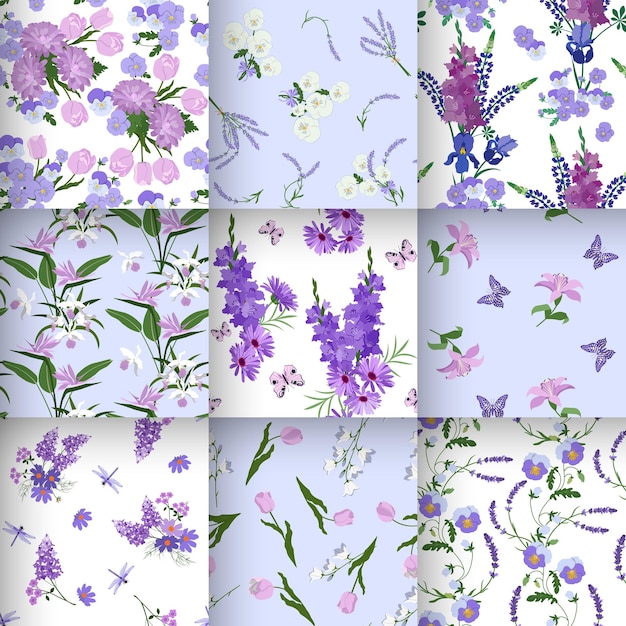The image is a collage of nine individual square photos arranged in a 3x3 grid. Each square features an intricate design of flowers, predominantly in pastel shades of light blue, light purple, and lavender. The backgrounds vary, with some featuring a soft powder blue and others a delicate white. Among the flowers, lilacs and lilies are prominent, adorned with green leaves and stems. The middle-right photo showcases purple butterflies fluttering among pink flowers, while the bottom-left square depicts blue dragonflies amidst lavender and other purple flowers. The top-right square contains darker blue and purple flowers. The overall theme exudes a serene, floral ambiance, accentuated by the consistent use of pastel colors and delicate botanical elements.